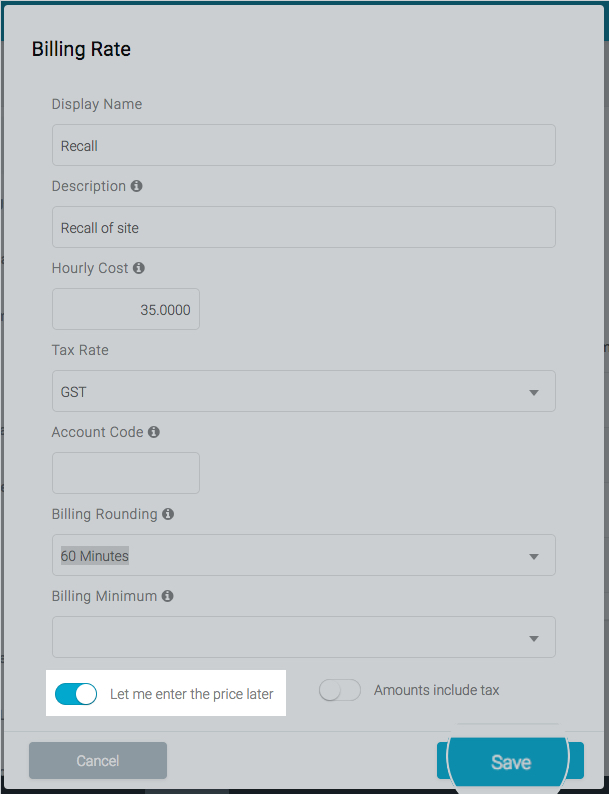This image is a screenshot taken from a website featuring a box titled "Billing Rate." The title is located at the top left corner, written in bold black text. Within this box, there are several fields and options arranged in a vertical list:

1. **Display Name:** A rectangular input field for entering the display name.
2. **Description:** Another rectangle for filling in a description.
3. **Hourly Costs:** This field is already populated with the value "35.0000".
4. **Tax Rate:** Labeled as "GST."
5. **Account Code:** This input field is currently blank.
6. **Billing Rounding:** This option is set to "60 minutes" and is highlighted.
7. **Billing Minimum:** This field is also empty.
8. **Enter the Price Later:** This toggle button is switched on.
9. **Amounts Include Tax:** This toggle button is switched off.

At the bottom of the box, there are two buttons: a "Cancel" button on the left and a "Save" button on the right.